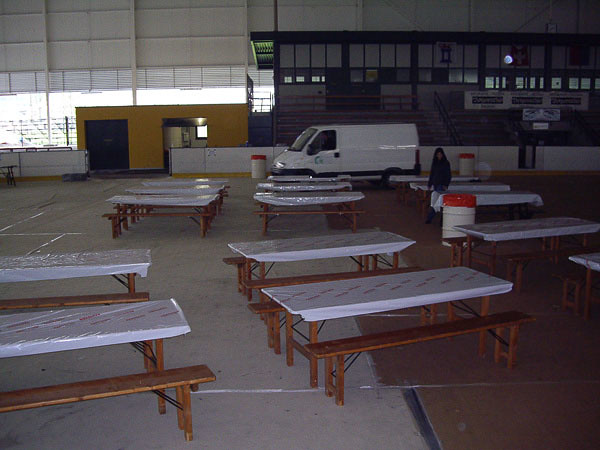The image shows the interior of an ice hockey stadium being prepared for an event, possibly a picnic or luncheon. The central area, which features boards typical of an ice rink, holds approximately 13 to 14 rectangular picnic tables made of wood, each draped with a white tablecloth adorned with red lettering. The left side of the floor appears icy, while the right is covered with cardboard. A white utility van is parked toward the rear. In the background, the stadium stands can be seen, along with various signage and a yellow area with a blue door, possibly leading to restrooms. Three barrel trash cans with white bases and red bags are positioned among the tables. One person, likely female, wearing a dark-colored shirt and with dark hair, is visible. The setting is indoors with some daylight filtering through, giving a dark and shady ambiance. The overall scene suggests a setup for a food-related activity in a spacious, multi-functional indoor arena.